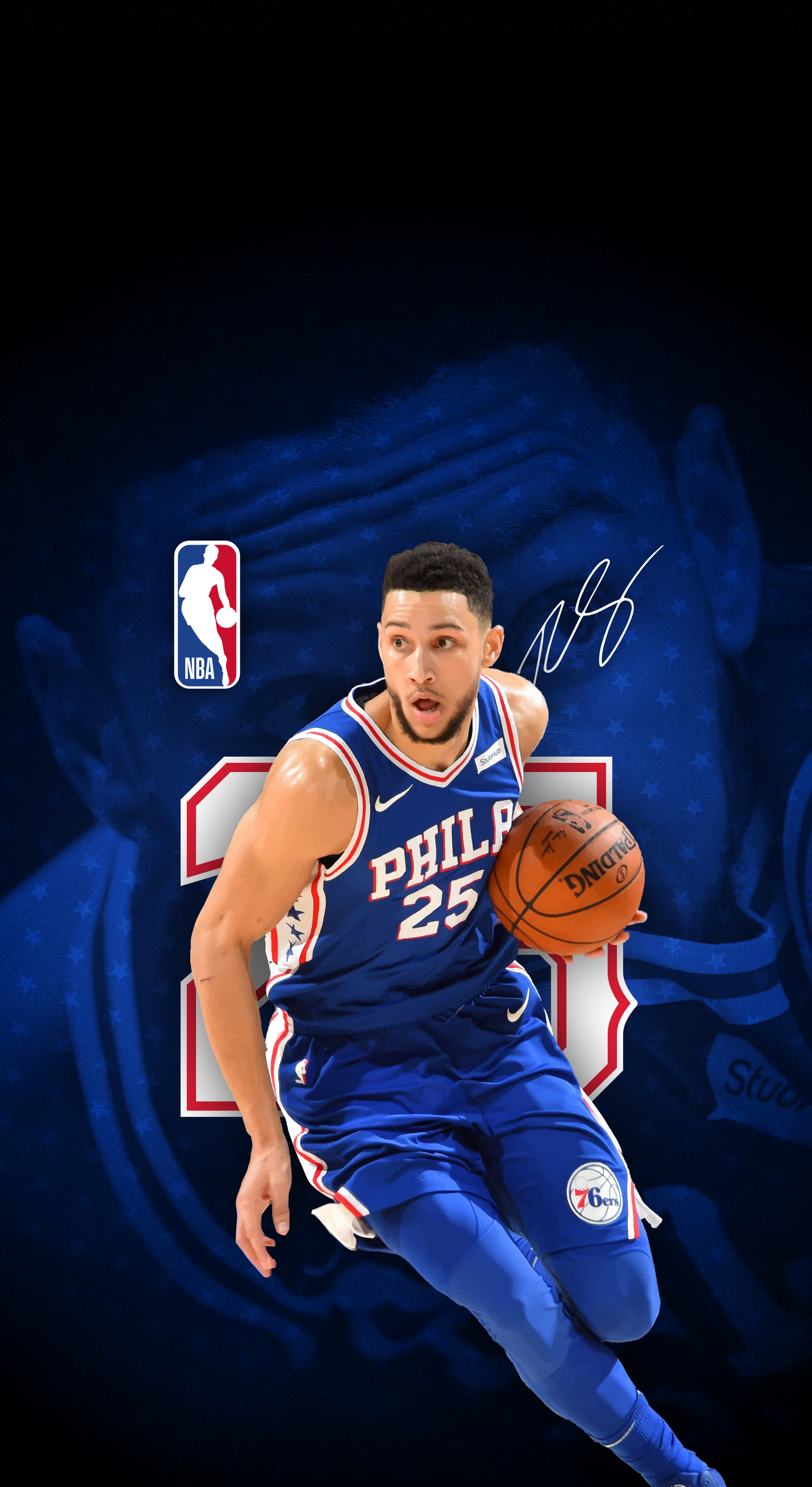This image is a digitally illustrated color photograph of a professional basketball player named Philip, a member of the 76ers, wearing a complete blue uniform. His attire includes a blue Nike jersey emblazoned with his number, 25, in white text, along with the Nike Swoosh logo on the top left corner and the NBA logo positioned in the upper left of the image. He is also equipped with matching blue shorts, blue leggings, and blue sneakers, completing his team outfit. Philip, with short curly brown hair, a light mustache, and a beard running along his jawline, is captured in mid-motion, clutching a Spalding basketball in his left hand as though contemplating his next move. His right hand hangs down by his side, and he is depicted mid-stride, with one foot lifted. The background has been digitally altered to be entirely black, with an additional blue-toned close-up of Philip’s head and his number subtly rendered behind him. His messy white signature is also visible next to his face, adding a personal touch to the image, which might be utilized as a trading card or a poster.